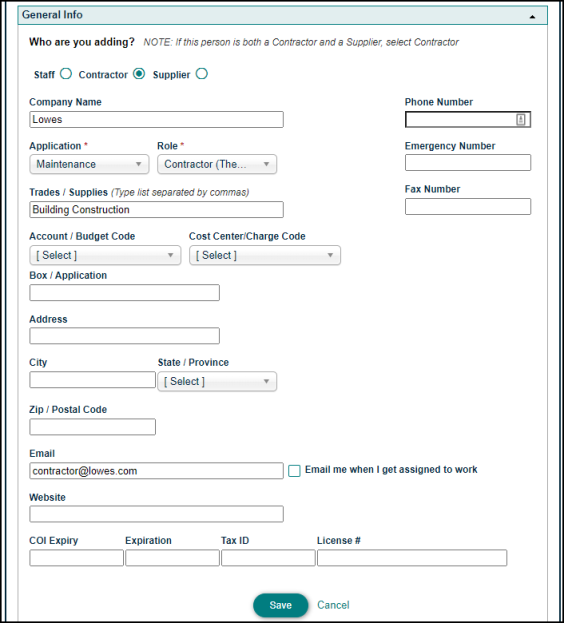The image is a vertical screenshot from a website, framed by a black border with seafoam green teal lines running down the left and right sides. Across the top, there is a light blue rectangular box. In the upper left-hand corner, the text "General Info" is displayed, followed by a bold heading that reads "Who are you adding?" Below this, in lighter black or gray text, it states, "Note: if this person is both a contractor and a supplier, select contractor."

There are options presented to select roles, with the "Contractor" option selected. Other roles include "Staff" and "Supplier." The company name field is filled in with "Lowe's." Additional fields include "Phone Number," with sub-labels such as "Application Maintenance Role," marked as "Contractor," and an "Emergency Number" field which is not filled in.

The "Trade Supplies" entry box lists "Building, Construction," separated by commas, though not all supply types are selected. The "Account Budget Code," "Cost Center," and "Charge Code" fields prompt the user to press "select" as they are still blank. Address details such as "Address," "City," "State/Province," and "ZIP/Postal Code" are also not filled in. The email field contains "contractor@lowes.com," with an option to check a box labeled "Email when I get assigned work," which is currently unchecked.

Fields for "Website," "COI Expiry," "Tax ID," and "License Number" remain unfilled. At the bottom, there are buttons for actions: a seafoam green "Save" button and a "Cancel" button.